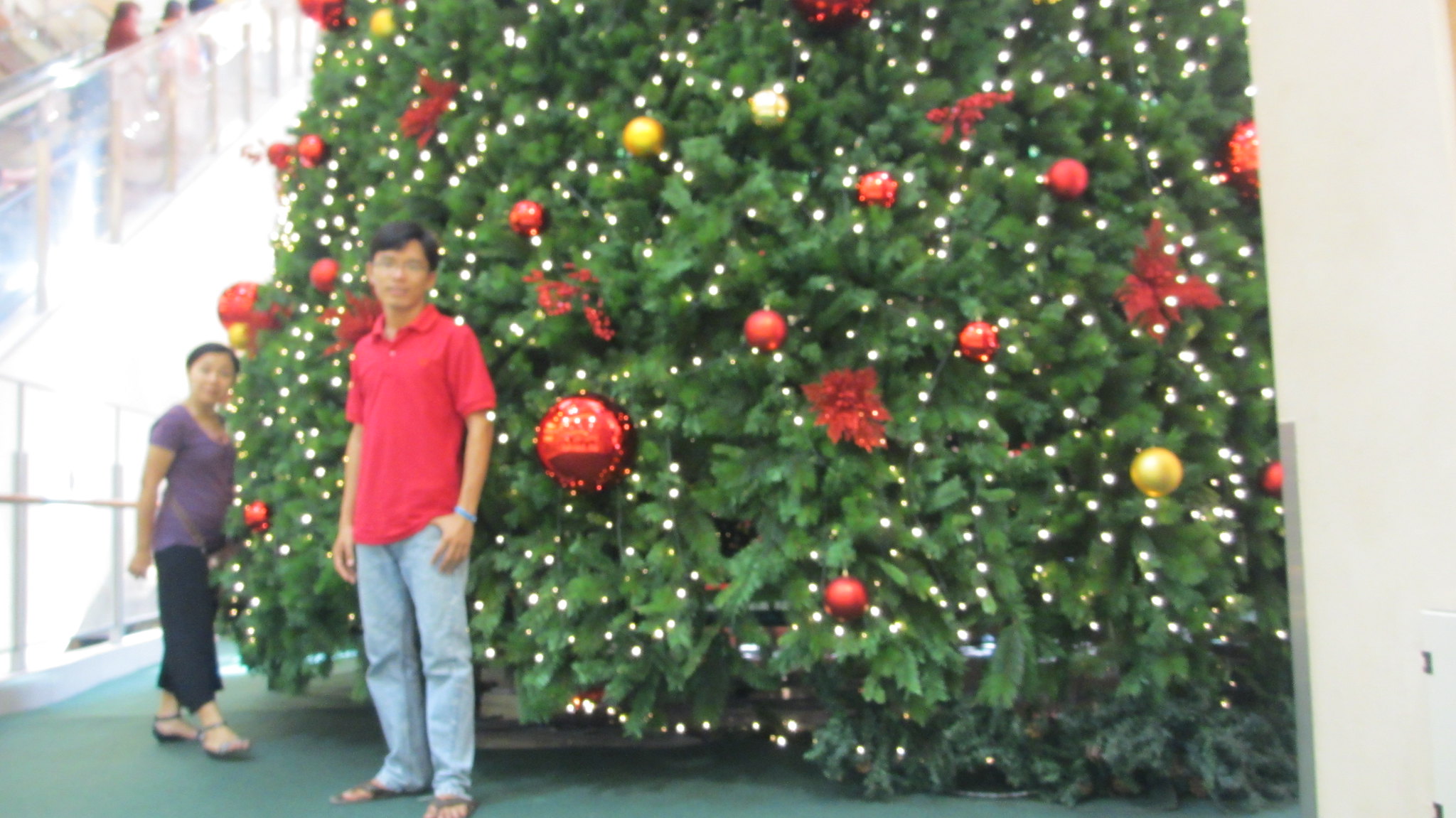The photograph captures two people standing in front of an enormous Christmas tree, set within a significant indoor space, possibly a convention hall or a large building with what appears to be a balcony floor. The tree, adorned with numerous small white lights and a plethora of ornaments in various sizes and colors—including shades of red, gold, and silver—is partially obstructed by a column, with its full height cut off around 12 feet from the base. To the left, a section of glass showcases an upper floor with people standing, and there is also an escalator or stairway visible, suggesting the grandeur of the space.

The man is dressed in blue jeans and a red polo shirt, while wearing glasses, and the woman is clad in a blue short-sleeved shirt and black capris. Both are sporting sandals. The decorations also include red bows, adding to the festive appearance. Despite the photo being slightly blurry, the width of the tree, estimated to be at least 20 feet, and the lavish decorations make it a spectacular sight.